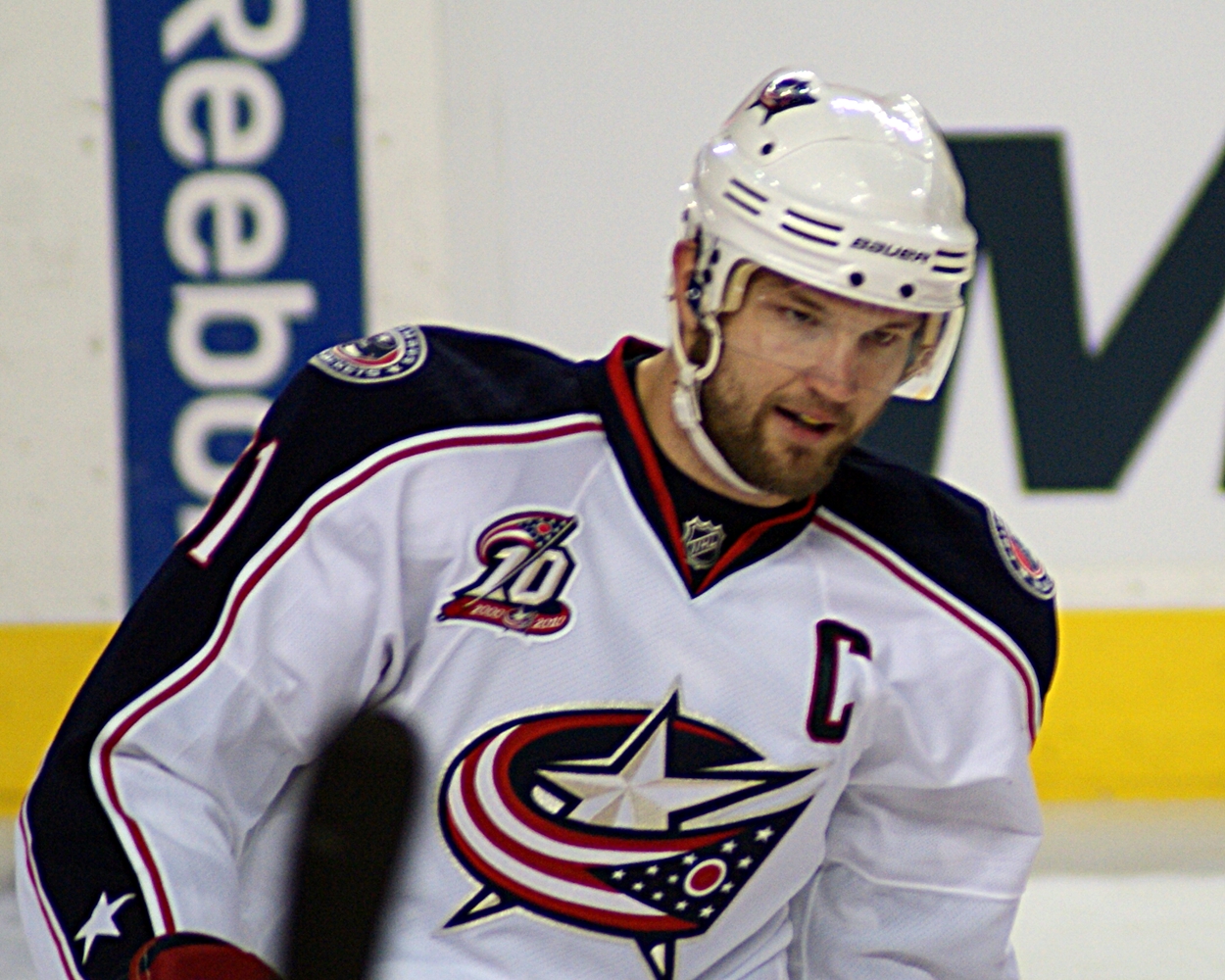The image depicts a white background with a blue rectangular shape prominently featuring the partial text "EBOC," suggesting a Reebok advertisement. Additionally, a black letter "M" appears partially cut off on the right side, set against the backdrop with a yellow stripe at the bottom, all situated on what seems to be an ice hockey rink. 

In the foreground stands a white male ice hockey player, captured from head to waist. He has brown eyes, a reddish-brown beard, and a moustache. He wears a white or cream-colored protective helmet with a plastic shield covering his eyes and a securing strap under his chin. His body tilts slightly to the right. 

The player dons a white jersey featuring a logo with a five-point star and a red and white swirl. On the left side of his chest, there's a 'C' indicating his captaincy, an American flag, and the number 10. His right shoulder displays a patch, and blue stripes run down both shoulders, while black blocks extend down the arms. The overall scene suggests he's part of a team, possibly the Capitals, engaging in an ice hockey game.